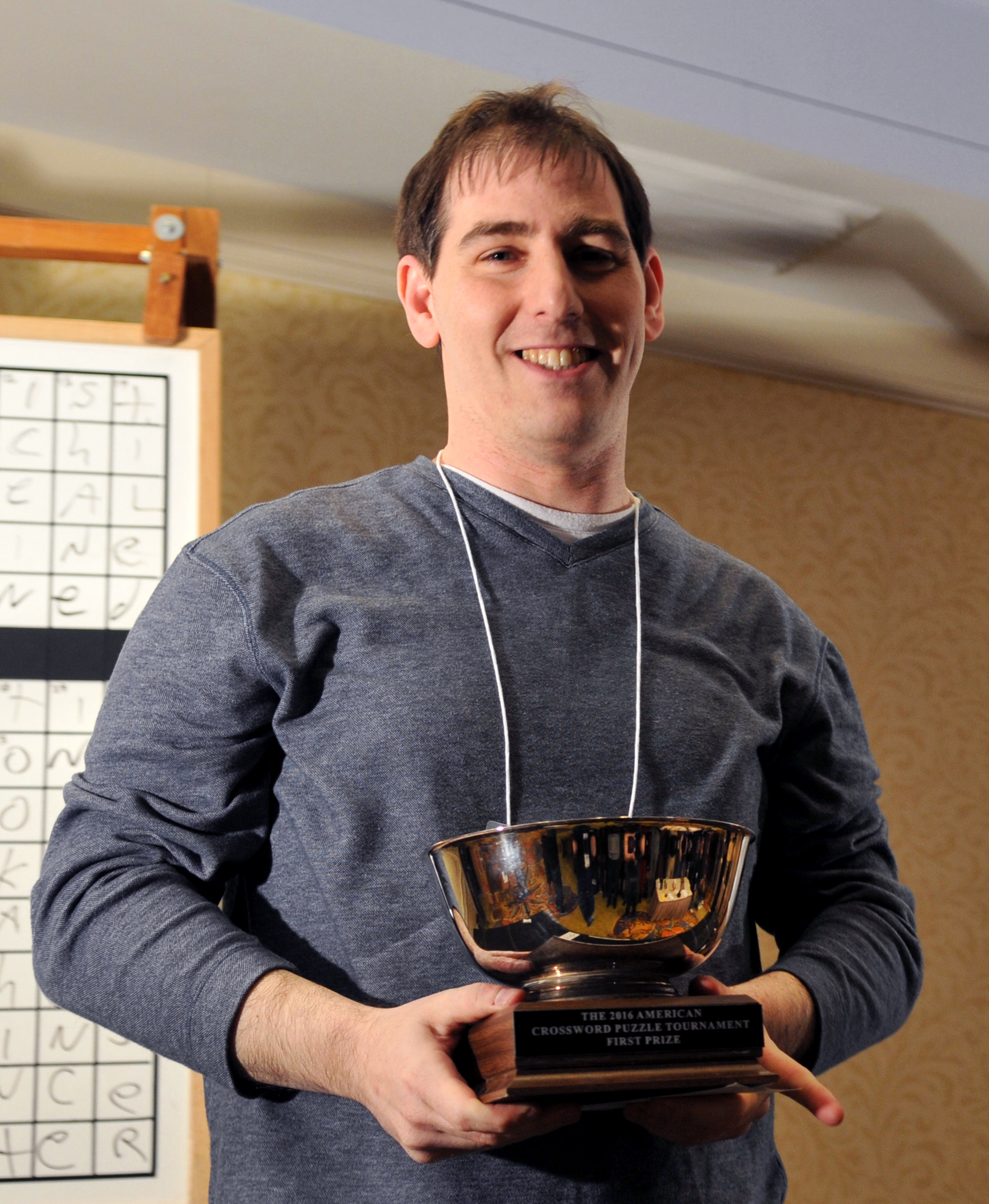This is a detailed color photograph of a young man with short dark hair, smiling broadly and looking directly at the camera, his eyes slightly cast downward. He is holding a large trophy with a wooden base and a gold bowl on top, in both hands. The trophy's plaque reads "2016 American Crossword Puzzle Tournament First Prize." He is wearing a grayish-blue long-sleeved shirt with a slight V-neck, over a white undershirt, and his sleeves are rolled up. Around his neck hangs a white cord, likely attached to a name tag. Behind him is a textured tan wall with a darker tan pattern and a whiteboard with a handwritten completed crossword puzzle. The room is dimly lit, casting a shadow on the ceiling.